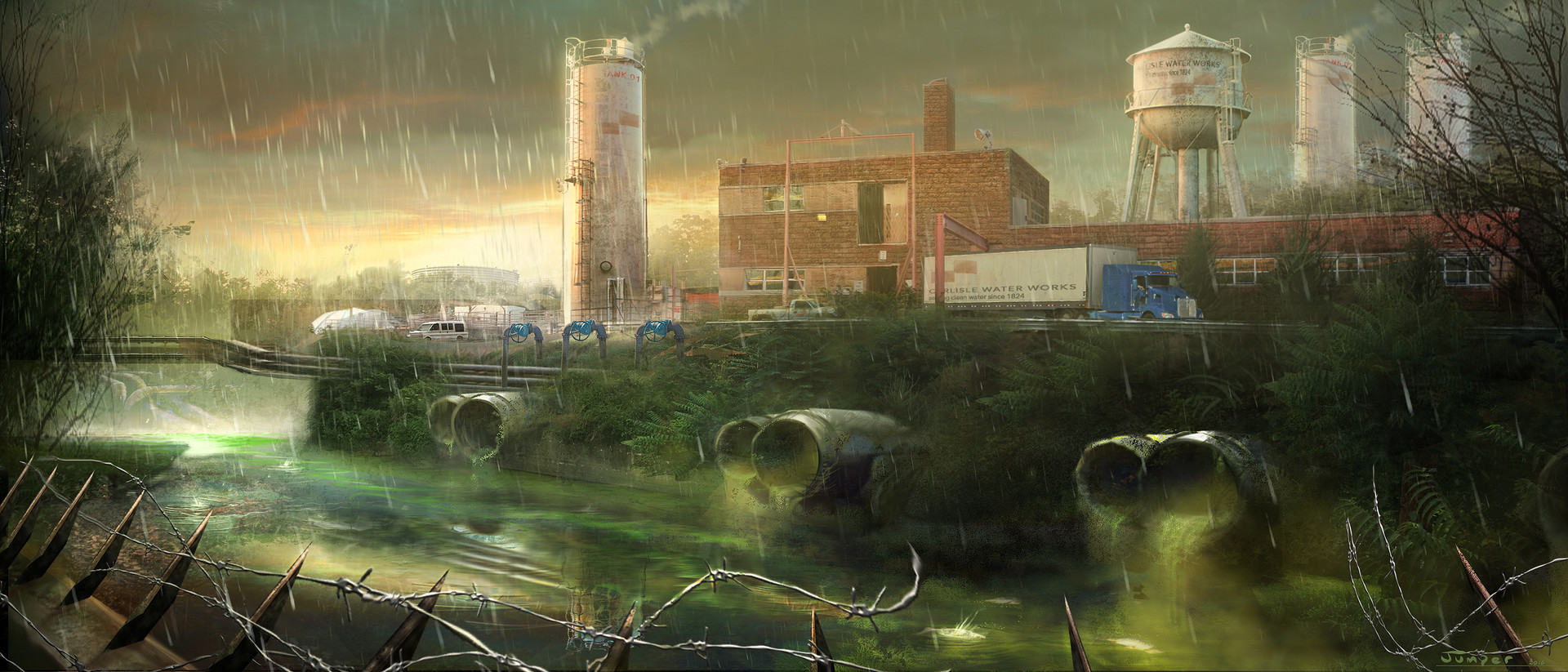This vividly detailed color illustration, possibly an oil painting or a digital creation, showcases a grim outdoor scene in an extreme, nearly rectangular, landscape layout. Dominating the upper right quadrant is a sprawling water treatment plant with various industrial structures. Central to the scene is a towering white structure exuding white smoke, alongside a reddish-brown, two-story brick building with an exhaust chimney and a white water tower supported by vertical posts. Further to the right, two more cylindrical white towers emit smoke into the murky atmosphere.

In the immediate foreground, a low-lying brick building is fronted by a massive tractor-trailer truck with a blue cab and a white bed, alongside a striking red object. The truck is parked on a grassy bank that slopes downwards towards a river or stream, characterized by its toxic appearance with green and yellow hues.

Six large silver pipes protrude from beneath the building, spewing a luminescent, lime-green, smoky liquid into the water below. This stream, curving leftwards, is enshrouded in an ominous green haze. Above, a stormy sky looms with dark, rain-filled clouds, adding to the dreary atmosphere. In the lower left corner, a dilapidated barbed wire fence further accentuates the desolation of the scene. The bottom right subtleties include a barely discernible signature, hinting at the artist's identity.

This compelling composition, with its fantasy-like elements and stark depiction of pollution, invites viewers to ponder the environmental impacts of industrial activities.